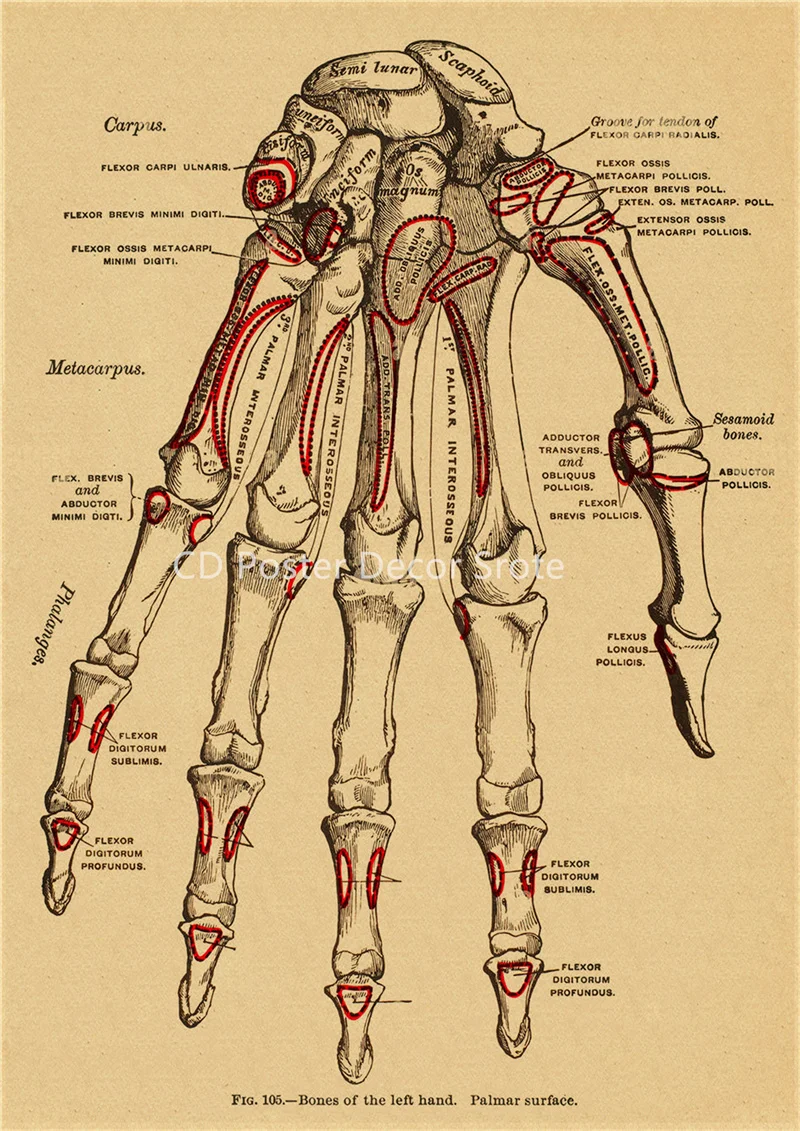This detailed anatomical drawing illustrates the skeletal structure of what appears to be a human right hand, oriented with the wrist at the top and the fingers pointing downward. The bones are meticulously rendered, with various sections highlighted in red ink to emphasize specific areas. Surrounding the hand, tiny print labels all of the different bones and sections, presumably discussing their names and characteristics, though the text is too small to be easily readable. The bottom of the image is marked with the title "Figure 105 - Bones of the Left Hand, Palmar Surface" in black lettering, and the middle of the hand is overlaid with the text "CD Poster Decor Store" or something similarly phrased. Although the accompanying notes appear to be written in Latin, enhancing the scientific precision of the illustration, they provide detailed descriptions of intricate bone structures like the flexor digitorium sublimus and semoid bones.